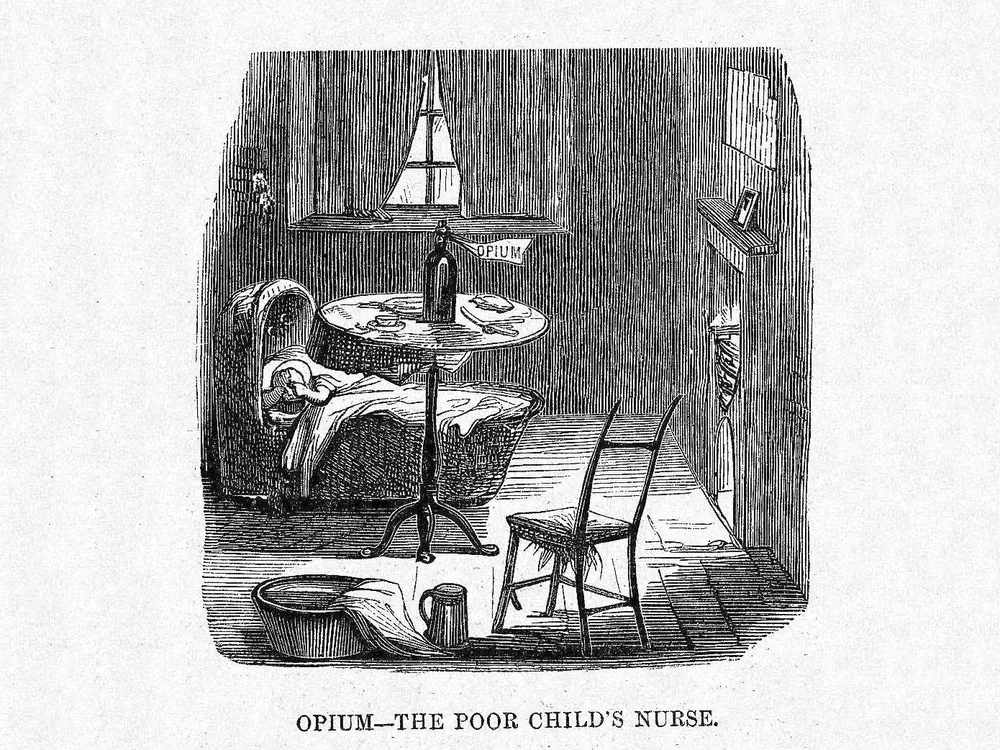This black and white line drawing, reminiscent of a children's book illustration, appears to be an illustrated advertisement or political cartoon on grainy white parchment. The scene is set in a dimly lit, small room dominated by a critiqued narrative evident in the text at the bottom that reads "Opium, the poor child's nurse." Central to the composition is a round, single-legged table holding a prominently labeled opium bottle with a cork and a flag attached to it. A baby rests in a hooded crib to the left, its face contorted with a hand on its forehead and another at its eyes, suggesting crying. The crib is draped partially with a blanket, and directly behind it, curtains obscure most of a window. On the right, a fireplace, the room’s primary light source, casts a warm glow. Near the table, there is a small wooden chair, and to its left, a washbasin with a towel hanging out and a metal pitcher nearby. Various items, including a plate and knife, clutter the tabletop, while a small framed picture sits above the mantle, completing this sobering tableau.